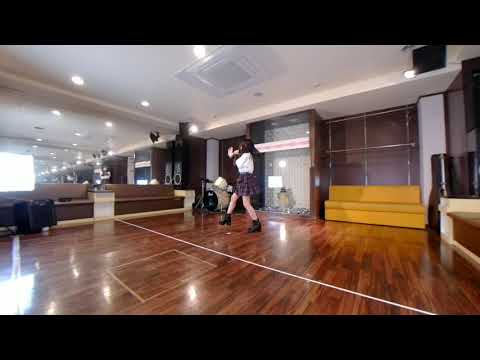The image showcases an indoor setting, likely a dance studio, characterized by solid black rectangular borders at the top and bottom. The center of the image features a shiny, reflective hardwood floor with a varnished wood grain finish. Centrally positioned is a young woman who appears to be dancing, wearing a skirt, boots, and a white top. She stands out as the focal point against the background of various objects. To the left, there's a large mirror and excellent recessed lighting in the ceiling. On the right side, a tan couch is visible, with more seating options spread throughout the room, including a yellow couch at the top center. Other elements in the room include what seem to be trophies and a drum set behind the young dancer. The overall impression is of a well-furnished room with vibrant colors like black, brown, white, light blue, yellow, pink, and purple, potentially serving as a versatile living space or a dance studio, captured in a somewhat pixelated image.